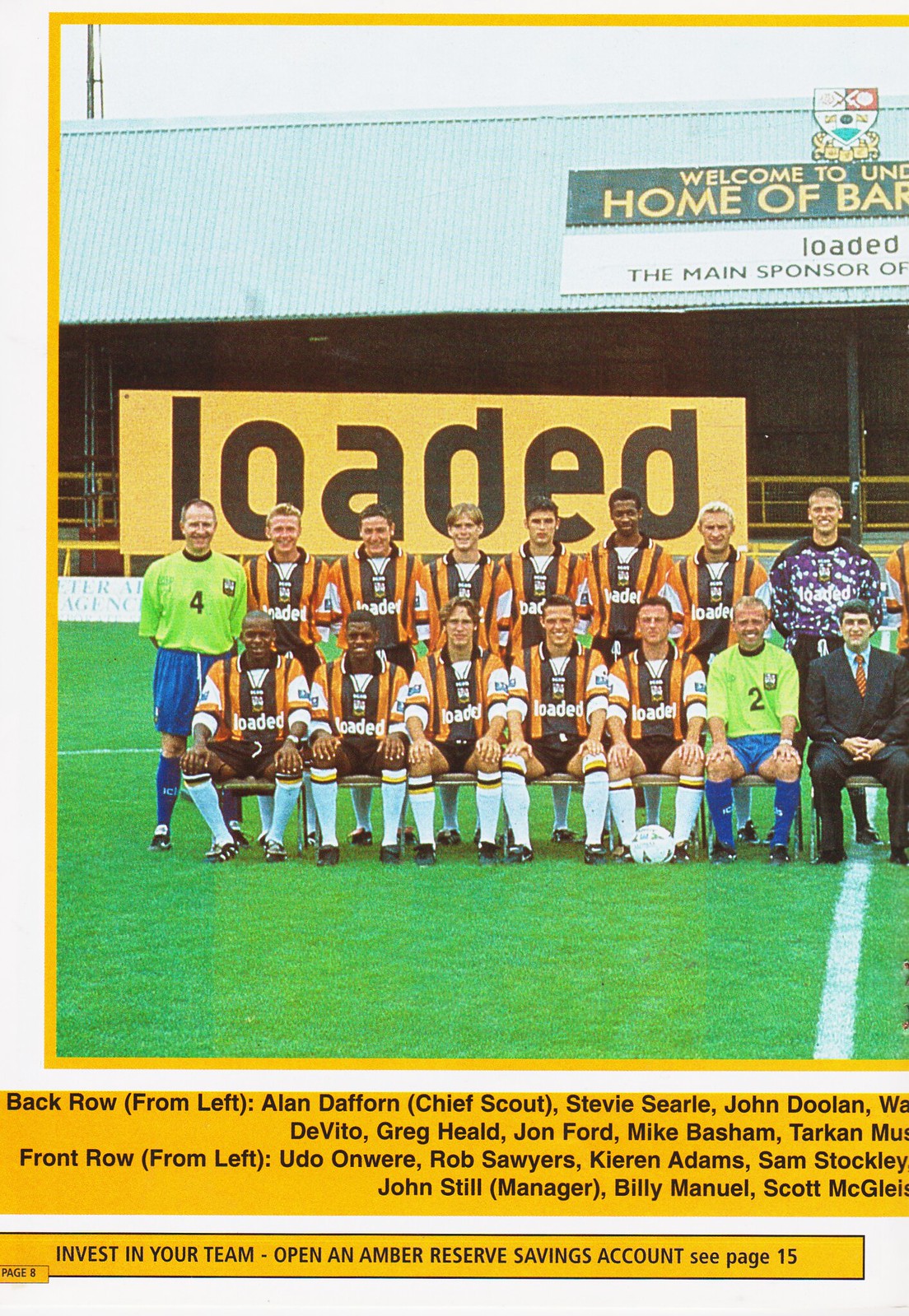This vertically-aligned, rectangular image appears to be a clip from an old newspaper article, possibly from the 1990s, depicting a children's soccer team. The photograph shows two rows of players and coaches seated and standing on a green field with white stripes, all in matching orange, black, and white uniforms, including knee-high white socks with orange and black stripes. A prominent sign in the background reads "Loaded" in large black letters on a yellow board. The team includes players of diverse backgrounds, and one seated player has a soccer ball positioned between his feet. Notably, two individuals, one on the far left and one on the bottom right, are clad in green and blue outfits, with the latter seated. Furthermore, there's a man in a suit and a man in a long-sleeve purple shirt with the word "Loaded" on it. The bottom of the image lists the names and titles of the team members and coaches, reading, "Back row from left: Alan Dafforn (Chief Scout), Stevie Searle, John Doolin, DeVito, Greg Heald, John Ford, Mike Bashman, Turcon. Front row from left: Udon Onware, Rob Sawyers, Kieran Adams, Sam Stockley, John Still (Manager), Billy Emanuel, Scott McLeish." The bottom text also encourages viewers to "Invest in your team. Open an Amber Reserve Savings Account."